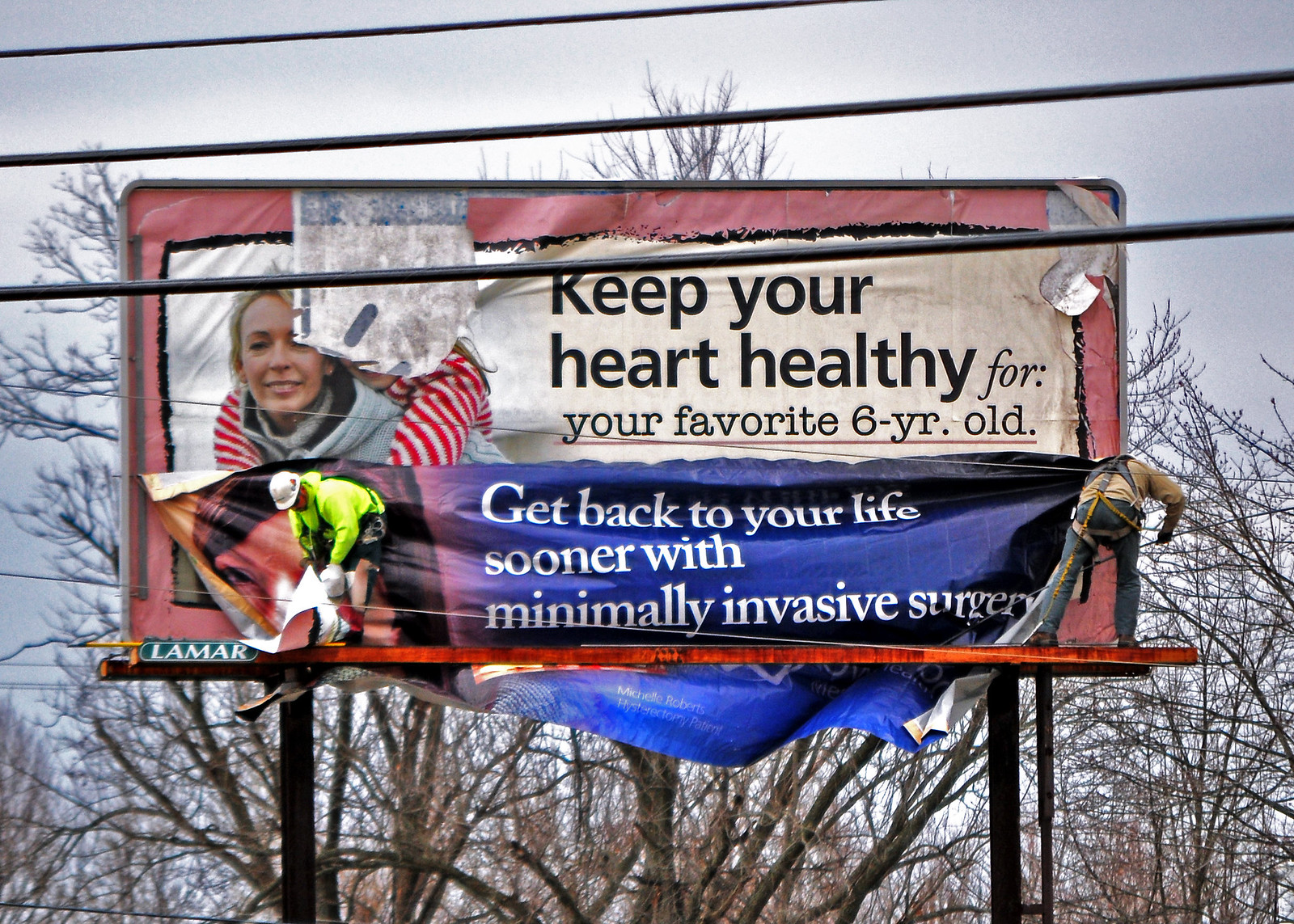A winter photograph showcases gray, somewhat cloudy skies with bare trees standing starkly in the background. In the foreground, seemingly captured from a highway, stands a large billboard with a notable pink background. The billboard's primary message reads, "Keep your heart healthy for your favorite six-year-old," accompanied by an image of a blonde woman carrying a child on her back. The child, donned in a red striped sweater, has their face partially obscured due to the billboard being partly torn away.

Adding to the scene's dynamic nature, two workmen are seen actively installing a new advertisement at the bottom half of the billboard. Positioned on either side, the workmen are attaching a segment featuring a woman's image on the left and a blue background on the right. Overlaying the blue area, white text declares, "Get back to your life sooner with minimally invasive surgery." The juxtaposition of the torn, weathered advertisement with the fresh, vibrant new one being affixed gives a sense of ongoing change and maintenance amidst a wintry, muted landscape.